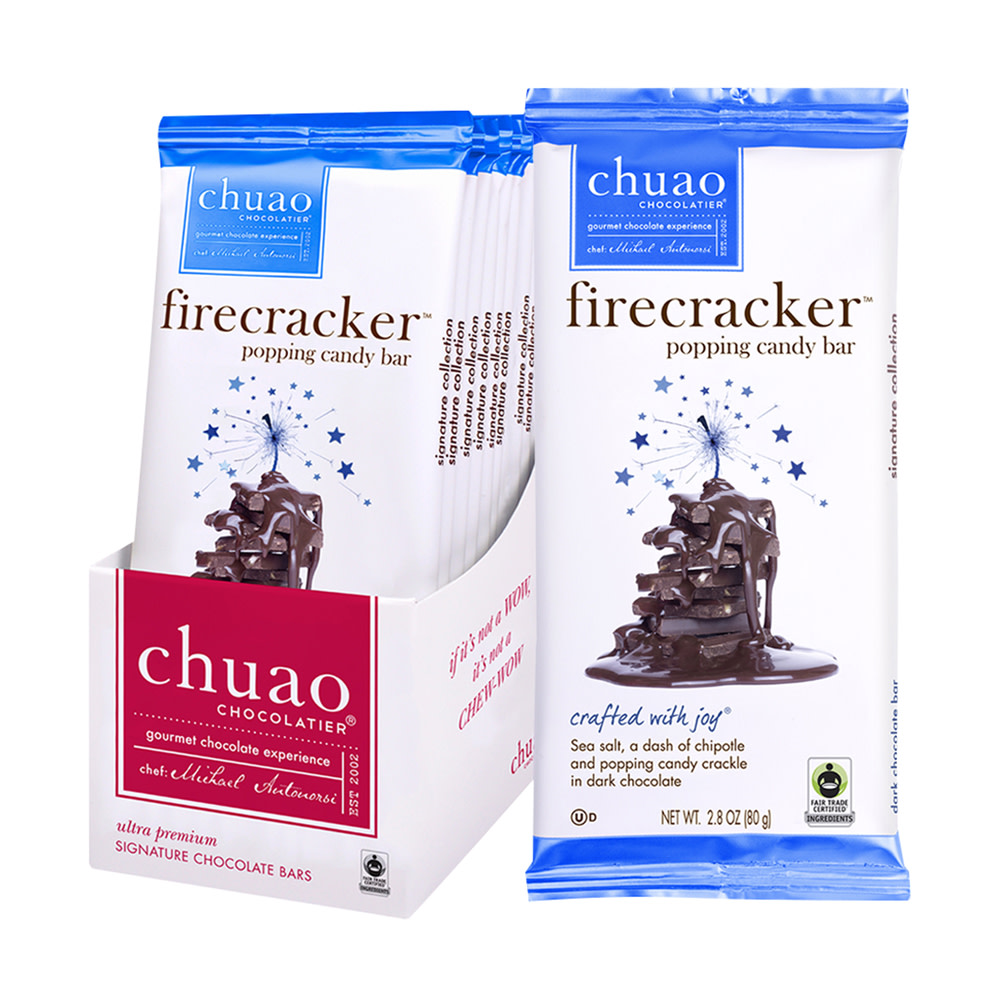The image is a detailed close-up photograph (stock photo) of a chocolate candy bar, prominently featuring the packaging of the "Firecracker Poppin' Candy Bar" by C-H-U-A-O Chocolatier. The entire wrapper of the candy bar is visible on the right side. The top part of the wrapper is bright blue, featuring the brand name "C-H-U-A-O Chocolatier" with the phrase "Gourmet Chocolate Experience" in white text. Below this, the wrapper transitions to white, highlighted by brown text that reads "Firecracker Poppin' Candy Bar." There's an illustration of a pile of chocolate pieces melting together, embellished with blue stars and a lit wake, symbolizing the popping candy effect. Further down in blue text, the wrapper describes the bar as "Crafted with Joy," containing "Sea Salt, a Dash of Chipotle, and Poppin' Candy Crackle in Dark Chocolate." The net weight indicated is 2.8 ounces. On the left side of the image, there are additional candy bars, partially visible inside a box, with a curved edge and red label that reads "C-H-U-A-O Chocolate, Ultra Premium Signature Chocolate Bars." The consistent blue highlights across the wrappers make the packaging visually striking and cohesive.